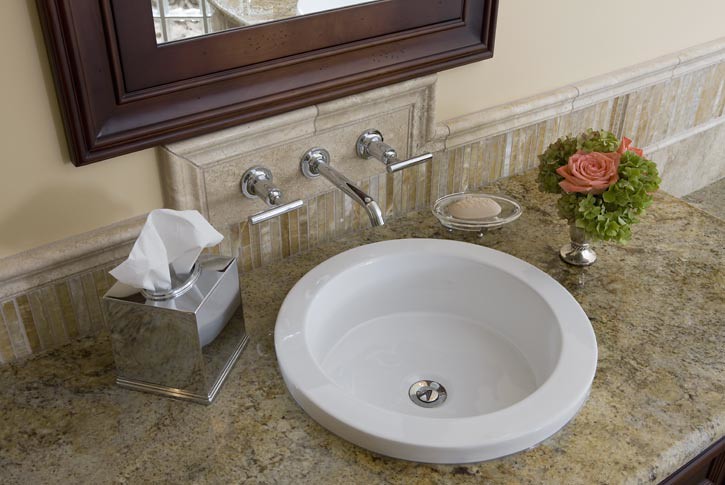The image depicts a meticulously designed bathroom counter. The backdrop consists of light beige walls adorned with elegantly arranged tiles. These tiles are segmented into smaller strips formed into larger blocks, each featuring a top trim piece that gives a neat finish. The countertop is crafted from granite, showcasing a blend of beige, dark brown, gold, and silver hues with a rounded edge, particularly visible at the lower right corner. 

A prominent feature on the counter is the round white sink. The sink has straight vertical sides with a relatively large rim that protrudes about one to two inches above the counter surface. Integrated into the wall above the sink is a sleek faucet with dual handles, one on the right and one on the left; both handles are flat bars in a polished silver finish. The sink’s basin includes a silver stopper, and the hint of water at the bottom suggests recent use.

Surrounding the faucet, the wall tiles extend an extra block above, framed with a decorative border, adding to the aesthetic appeal. Above this tile arrangement is a wooden-framed mirror with a distinctive scalloped design. The frame's contour includes two upward layers culminating in a curved edge, transitioning into a broad frame that narrows into a brown mat surrounding the reflective surface. The bottom of the mirror captures a faint reflection of the background tile work, adding depth to the scene.

On the left side of the sink sits a sleek silver Kleenex box, its white tissues peeking out from the top. To the right of the sink, closer to the wall, rests a crystal soap dish holding a beige bar of soap. Further right, a silver vase brimming with an arrangement of leaves and two pinkish roses is positioned, contributing a touch of natural elegance to the countertop setting.